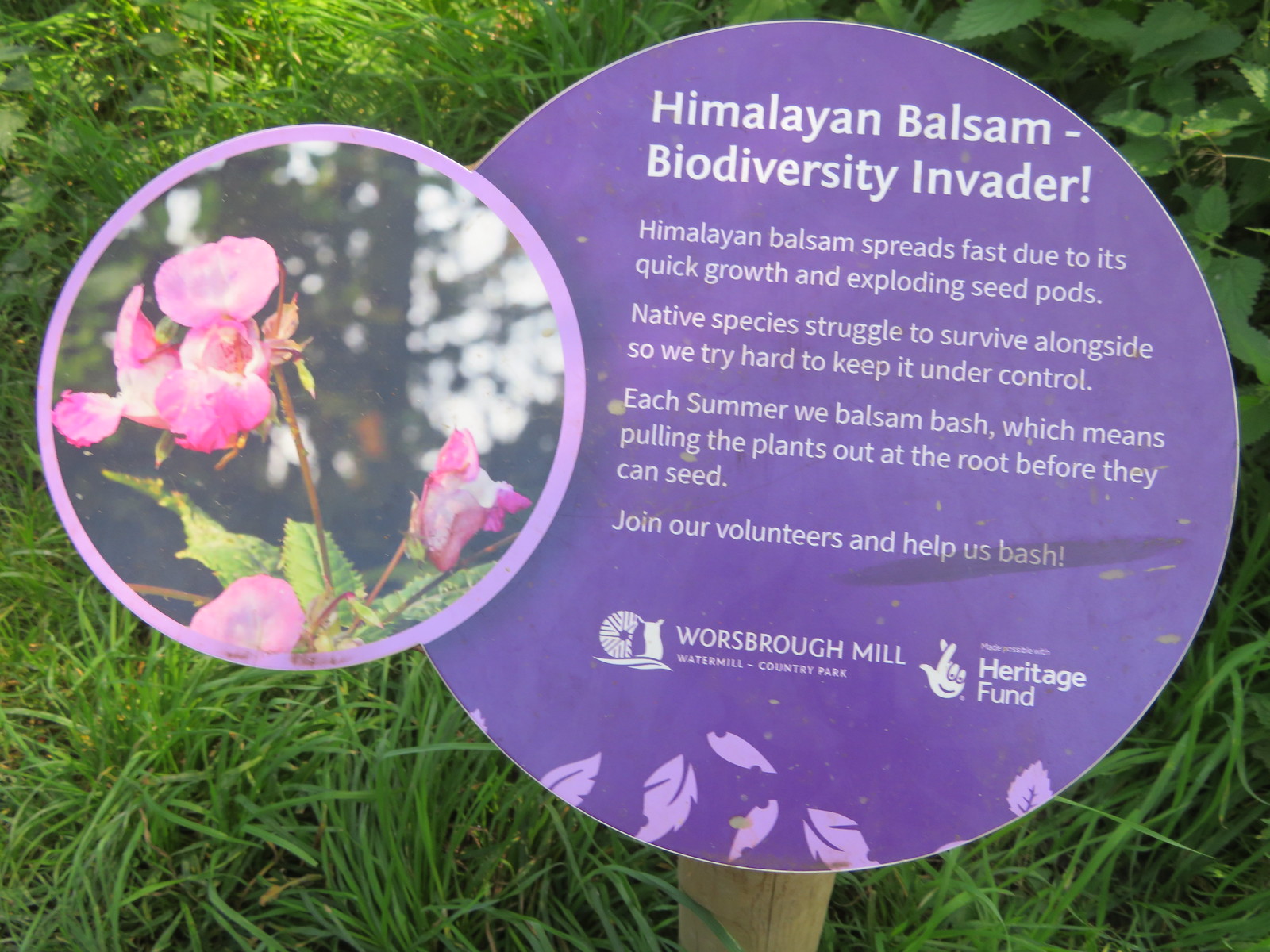In the image, a sign has been planted in front of a lush, green park or garden. The backdrop is full of long grass and leaves, creating a vibrant and natural setting. The main sign, which is bright purple with white text, stands out prominently. It is attached to another sign featuring pink flowers and additional green and brown hues. At the base of the main sign, cartoonish leaf designs add a playful touch.

The white text on the purple sign reads: "Himalayan balsam biodiversity invader. Himalayan balsam spreads fast due to its quick growth and exploding seed pods. Native species struggle to survive alongside, so we try hard to keep it under control. Each summer we balsam bash, which means pulling the plants out at the root before they can seed. Join our volunteers and help us bash."

The sign also displays logos for the Heritage Fund and Warsboro Mill Water Mill Country Park. The Heritage Fund logo depicts someone crossing their fingers, while the Warsboro Mill logo is less distinct, possibly resembling a slug.